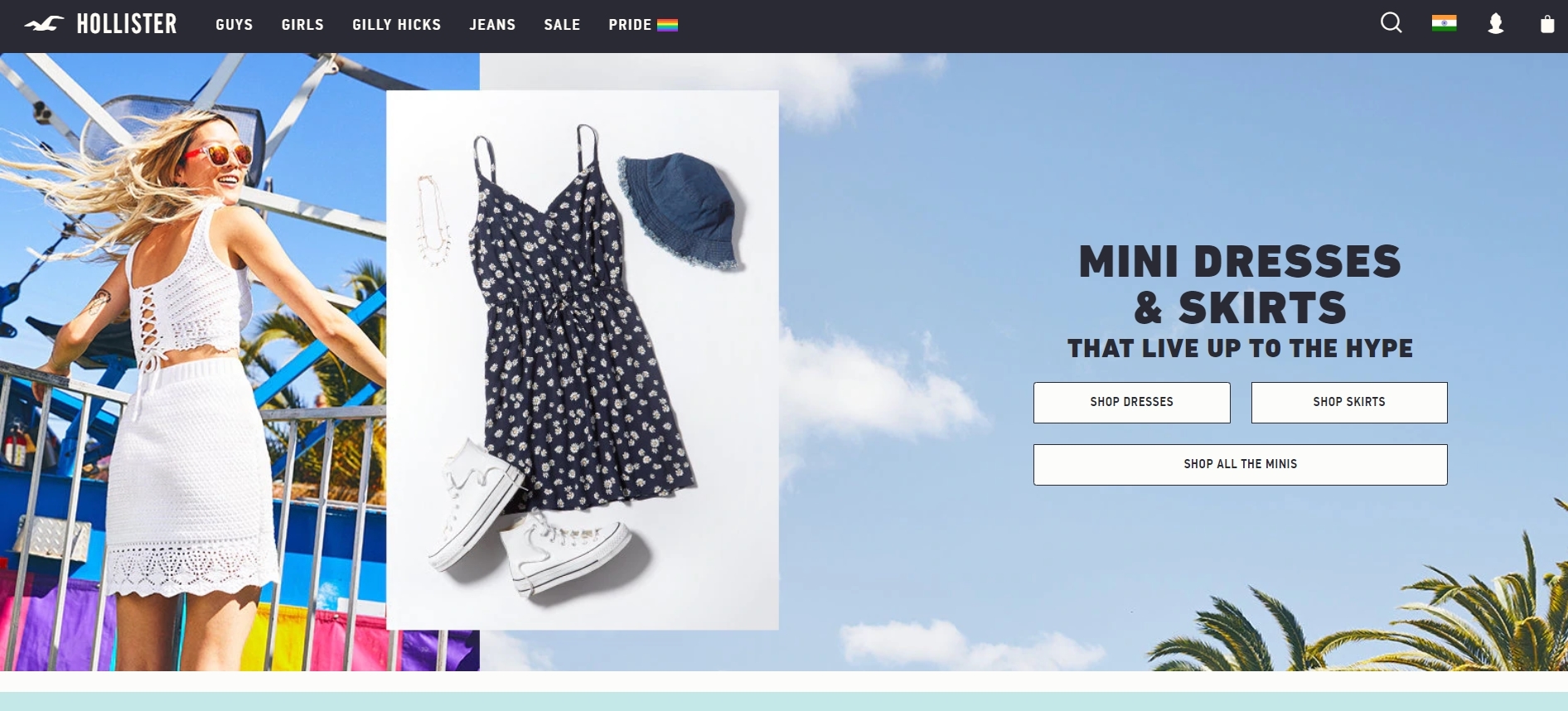At the top of the page, set against a sleek black background, is an advertisement for Hollister. The brand name "HOLLISTER" is prominently displayed in bold, white, all-capital letters, with their signature logo—a small white bird—situated to the left of the text. Below the brand name, the categories are listed in the same white, all-capital font: "GUYS," "GIRLS," and "GILLY HICKS," followed by "JEANS SALE" and "PRIDE." Adjacent to the "PRIDE" category is a vibrant rainbow flag. On the right side of the page, there are several icons.

Beneath this top section, the background transitions to a serene blue sky, adorned with palm trees. The central focus of the image is a blonde woman wearing glasses, a white tank top, and a white skirt. She is facing away from the viewer, her hair flowing behind her, as if she's gazing towards a Ferris wheel in the distance.

To the right of this scene is a vertical white rectangle showcasing a blue sundress with white designs, a white necklace on the left side, a denim pull-on hat on the right, and a pair of white high-top sneakers. This white rectangle is bordered on the right by another blue sky background with fluffy white clouds and the tips of palm trees in the bottom right corner.

The text "MINI DRESSES & SKIRTS" is prominently displayed in bold, dark letters, followed by the tagline "THAT LIVE UP TO THE HEIGHT" in slightly smaller, yet still dark and all-capital letters. Below this text are three clickable fields with a white background outlined in a dark color. They read: "SHOP DRESSES," "SHOP SKIRTS," and "SHOP ALL THE MINIS." 

At the bottom of the image is a small white area, under which lies a mint green horizontal rectangle.